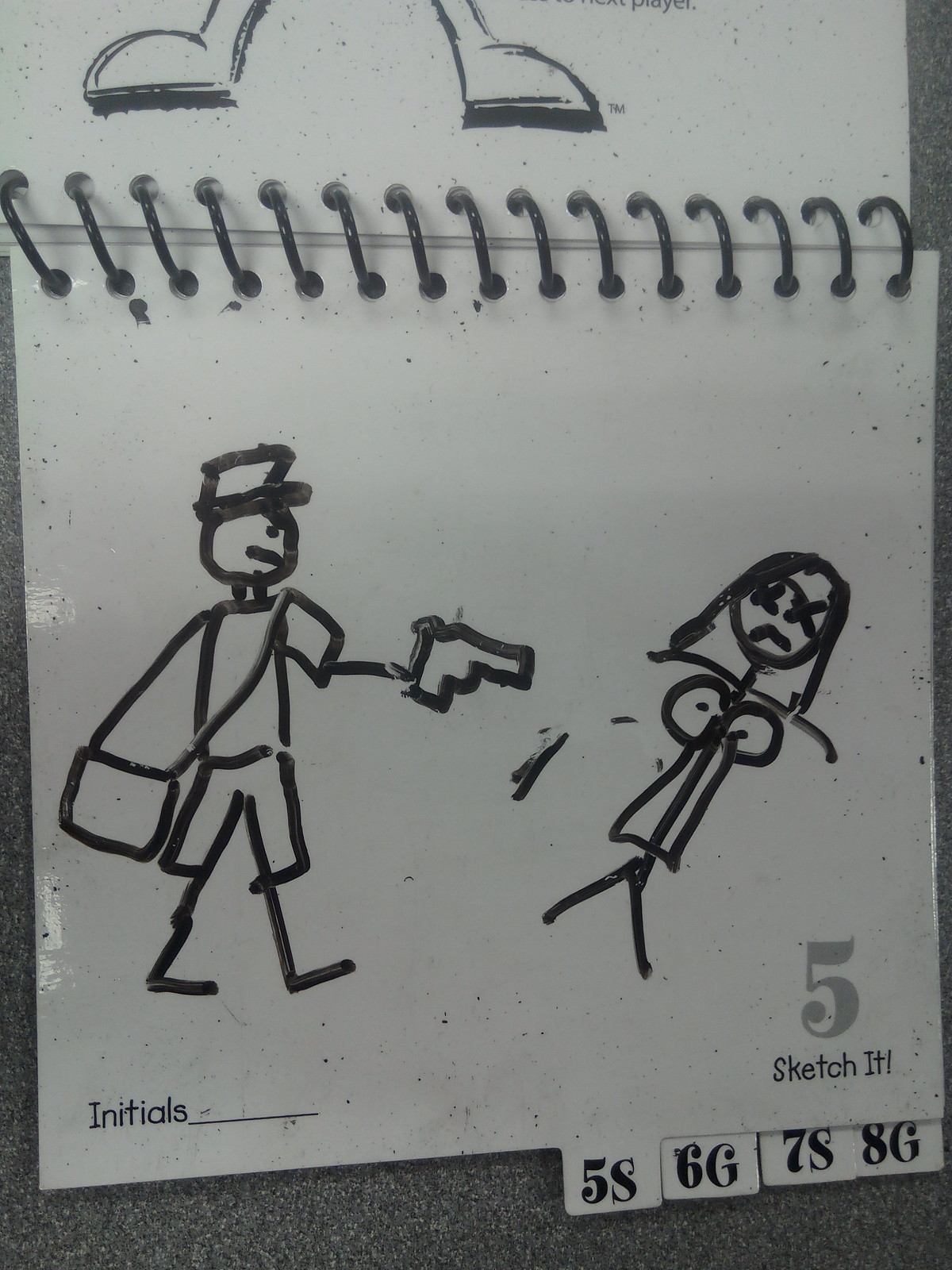The image is a hand-drawn sketch, created with a black dry erase marker in a spiral-bound sketchbook. The sketch depicts a rudimentary scene with two figures. The first figure resembles a mailman, characterized by a hat, a short-sleeved shirt, Bermuda shorts, and a satchel slung around the neck as a bag. This figure is holding a gun and aiming it at the second figure.

The second figure appears to be a woman, distinguished by exaggerated, large breasts, wearing a dress. Her face shows a distressed expression marked with X's in place of eyes and a pronounced frown. Notably, she seems to have no arms, with one area around her limbs showing signs of partial erasure.

In the background, the sketchbook’s details are visible, including the top spiral binding and a section for initials marked "5" with the phrase "Sketch it!" emphasized with an exclamation point. Tabs at the bottom of the page are labeled "5S," "6G," "7S," and "8G," suggesting organizational markers within the sketchbook.